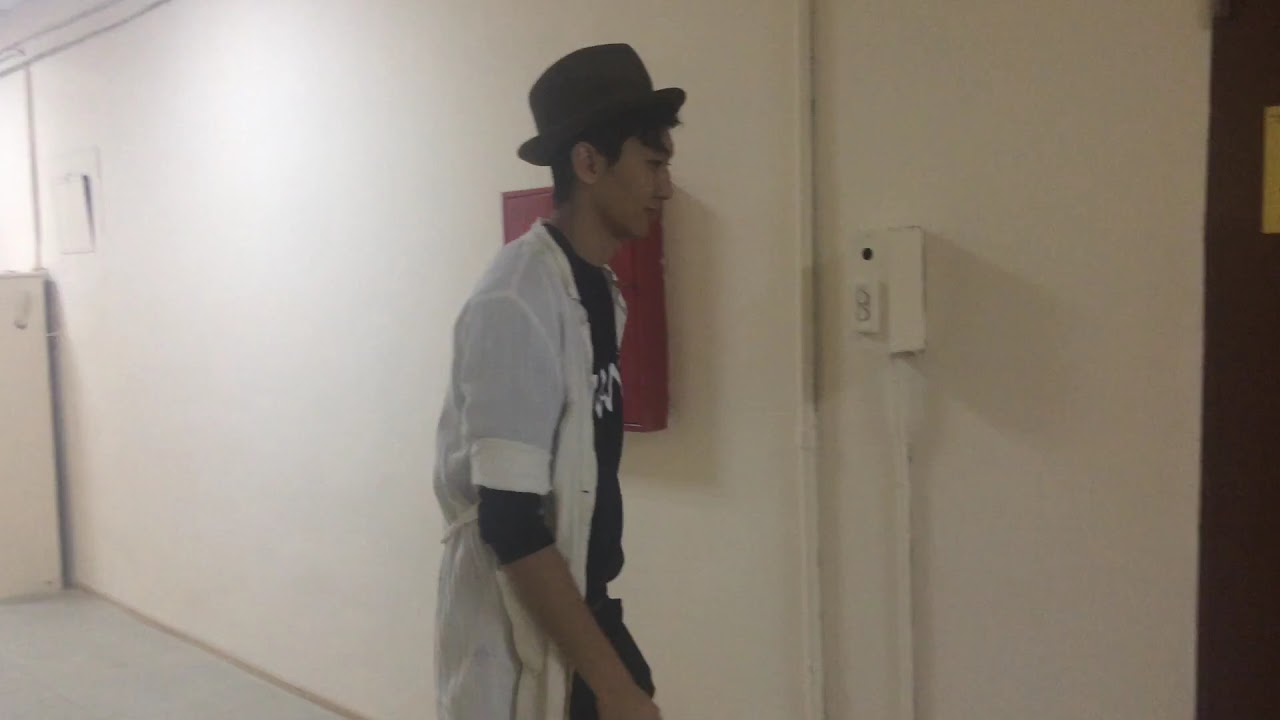The photograph captures a young, thin Asian man with no facial hair, standing in profile within a bright, white hallway inside a building. He sports a gray fedora over his short, dark hair and wears a white long-sleeve shirt, rolled up to the elbows, layered over a black t-shirt with indistinguishable white text. His right arm hangs at his side as he faces a wall to his right, where a dark entryway or door is partially visible. Directly behind him, affixed to the white wall, is a red emergency panel, likely for a fire alarm or similar device. To the right of this panel is some molding and an electronic device, possibly a phone or control box. The scene is lit by overhead fluorescent lighting, casting a uniform brightness across the white floor and walls.